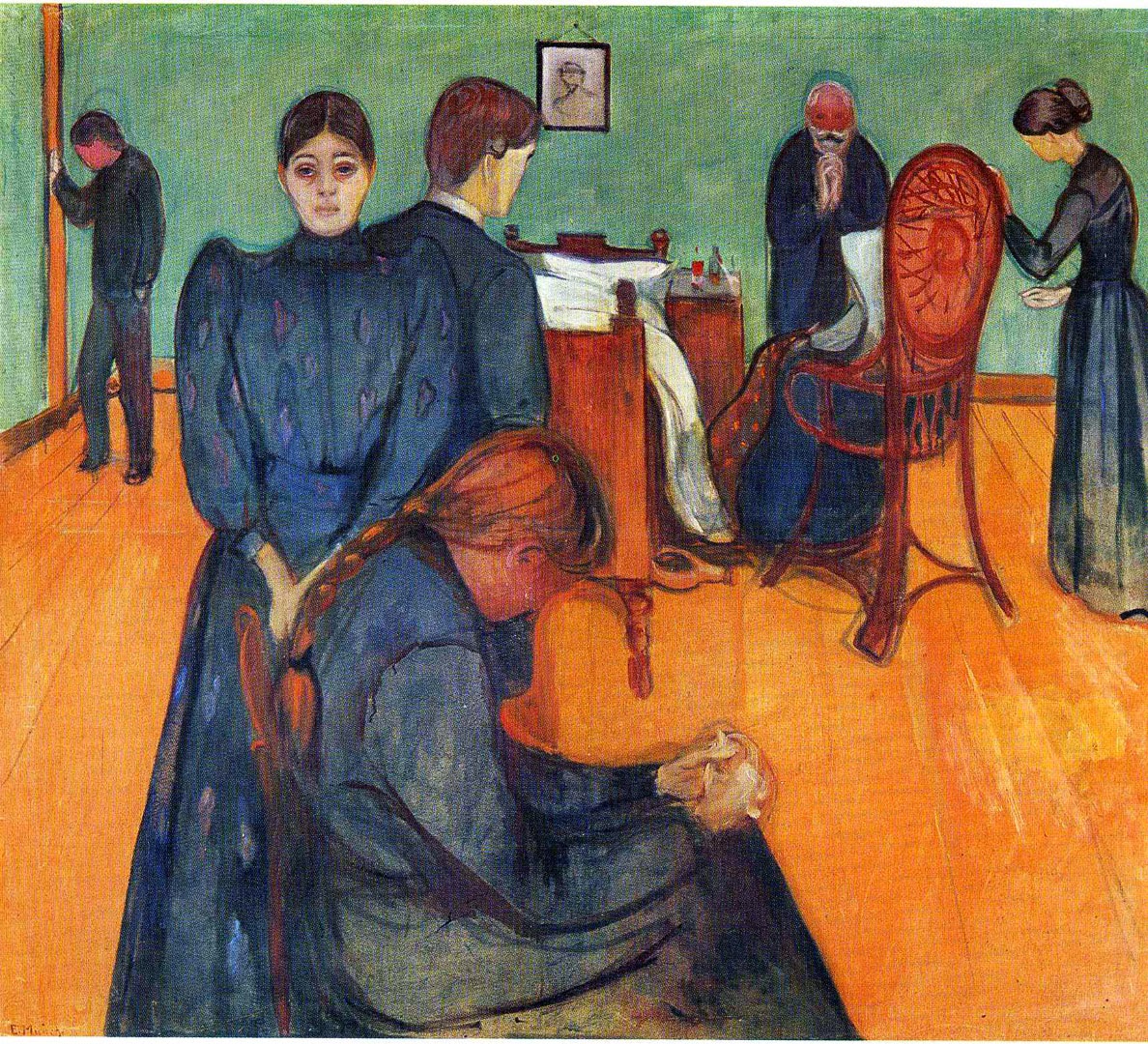This detailed painting illustrates an emotionally charged scene inside a room with green walls and an orange-brown hardwood floor. Central to the composition is a wooden bed draped with white pillows and blankets, above which a black-framed portrait hangs prominently on the wall. 

In the foreground, a woman with her hair in a long braided ponytail sits on a chair, hands clasped together in a prayerful posture. Directly behind her, another woman with an old-fashioned bun gazes into the camera, adding a direct emotional connection to viewers. To the left, a man is depicted in profile with his right hand extended to touch a vertical wooden beam, his head slightly bowed in deep thought.

To the right of the bed is a wooden chair facing away from the camera, occupied by an individual dressed in a dark outfit. In front of this person, an elderly man stands with his hands raised to his face in a prayerful gesture. Nearby, another woman rests her hand on the back of the chair, her dark clothing and solemn demeanor adding to the melancholic atmosphere.

The figures, all dressed in long-sleeved, dark blue or black clothing, contribute to the somber, reflective mood of the scene, resonating a sense of family or communal contemplation. Overall, the artwork, likely created with pastels, emphasizes themes of introspection and collective mourning.